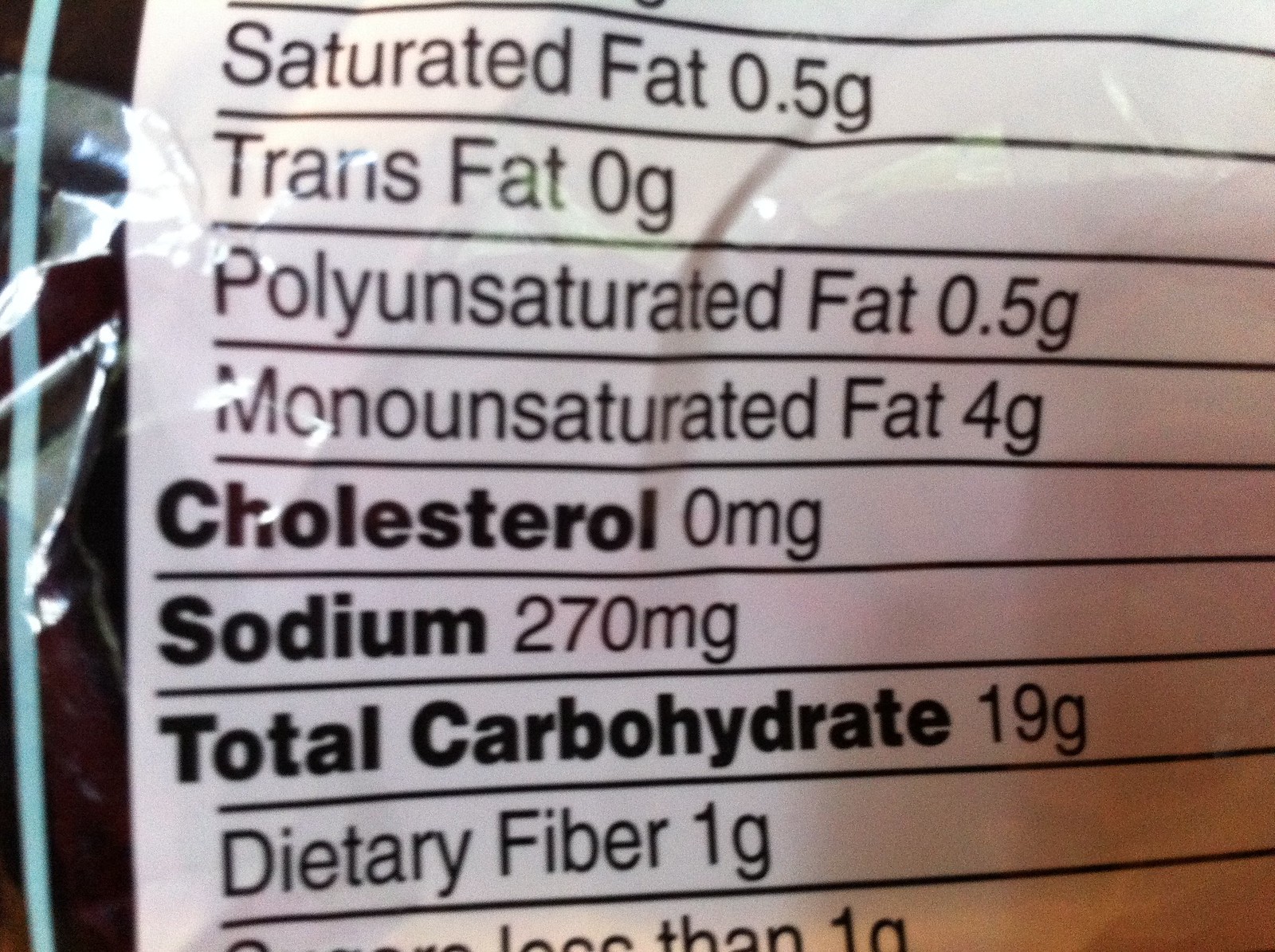The image depicts a highly magnified view of a nutrition label. At the very top of the label, the value for Saturated Fat is listed as 0.5 grams. Below this, the Trans Fat content is marked at 0 grams. Following that, the Polyunsaturated Fat content is recorded as 0.5 grams. Next, the Monounsaturated Fat content is shown as 4 grams. 

Further down, the Cholesterol content is emphasized in bold black text with a value of 0 milligrams (mg). Beneath this, the Sodium content is also highlighted in bold black text, with a value of 270 mg. The Total Carbohydrate content is bolded as well, marked at 19 grams. Below the total carbohydrates, the Dietary Fiber content is indicated as 1 gram. Unfortunately, the bottom portion of the label is not visible in the image.

All the nutritional values are presented in black horizontal text, with each section separated by a black horizontal line for clarity. The packaging appears primarily white but features a subtle light purple tint near the bottom. The left-hand side of the packaging is black, adorned with a light blue vertical stripe.